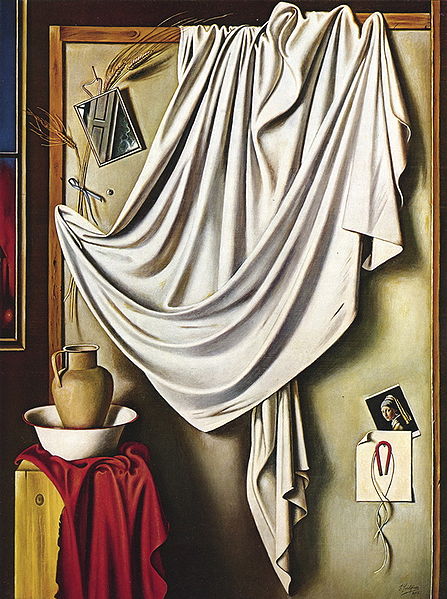The painting meticulously captures a scene centered around a large, brown wooden board with various objects meticulously arranged. Dominating the board is a vast white tarp or fabric draped over its front, partially covering the contents. On the top left, a piece of wheat is tacked, possibly with a mirror or a photo reflecting a door nearby. Multiple photographs and papers are pinned to the board, including a notable small image in the bottom right—a Polaroid-like picture of Vermeer's famous "Girl with a Pearl Earring," held by a pin with white string and a red hook.

To the left of this wooden board, there's a wooden table or stand, well-dressed in a rich red cloth. Atop this cloth rests a tan pitcher nestled inside a white wash basin. Slightly visible to the far left is a portion of a window, adding to the realism and depth of the scene. The overall composition and intricate details make it a striking, photorealistic depiction of an artful and thoughtfully arranged setting.